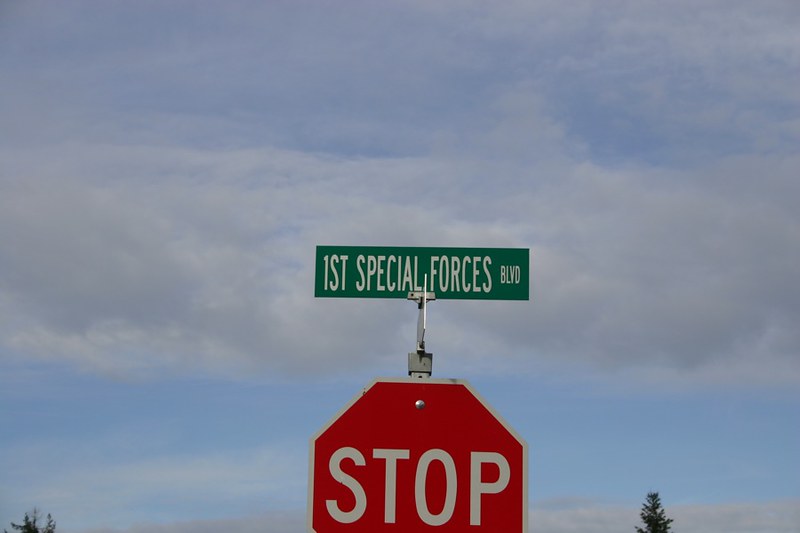The photograph captures the upper two-thirds of a traditional stop sign topped by a street sign against a serene backdrop of a partly cloudy blue sky. The stop sign is a classic red octagon outlined in white, with bold white letters spelling out "STOP." Above it, a rectangular green street sign with white lettering identifies the location as "First Special Forces Boulevard." The lower edge of the image reveals the very tops of two trees, suggesting the photo was taken from the base of the sign, angled upwards. The vibrant blue of the sky, dotted with wisps of cloud, contrasts with the rusty-red stop sign and the deep green of the street sign, while the patches of gray within the clouds and the greenery add subtle hues to the scene.